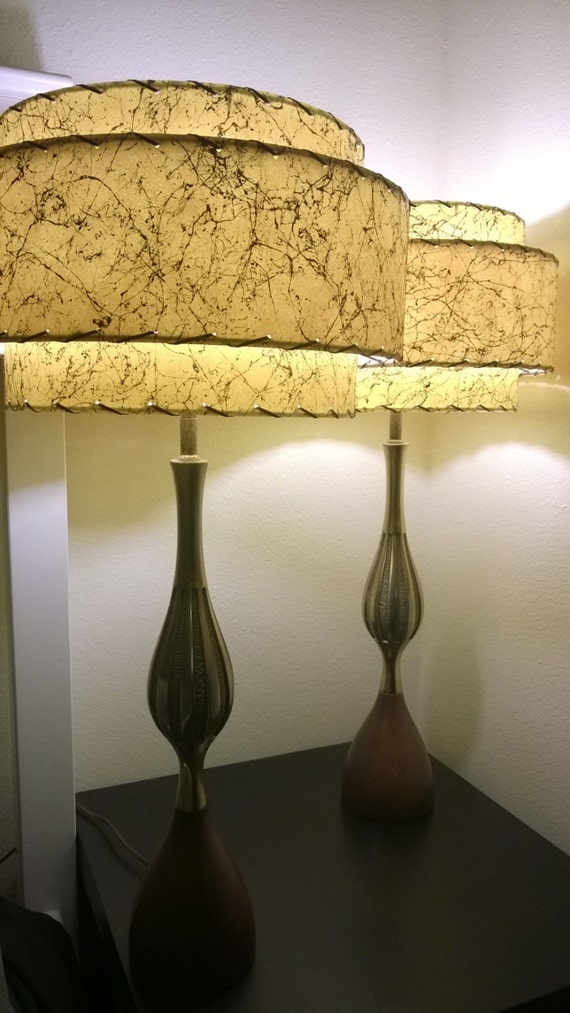This indoor image features two identical and unusually oversized lamps that capture attention with their distinctive design. The lampshades, which give the appearance of being made from paper, are a golden yellow color adorned with a black spackle or marbling effect that creates an intricate, web-like pattern. These drum shades have an outer layer and are finished with a laced-up edge around both the top and bottom. The lamps themselves have a sleek, tall structure with a bulbous, vase-like base crafted from metal and wood. These bases rest on a small, dark brown table positioned in the corner of a room, with a white, slightly textured wall as the backdrop. The setup includes a visible cable linking one of the lamps to a power source, illuminating the scene predominantly with the warm light from the lampshades. Off to the left, a white pillar can also be seen, adding to the overall setting. The lamps create a cozy and stylish ambiance reminiscent of 1970s decor.